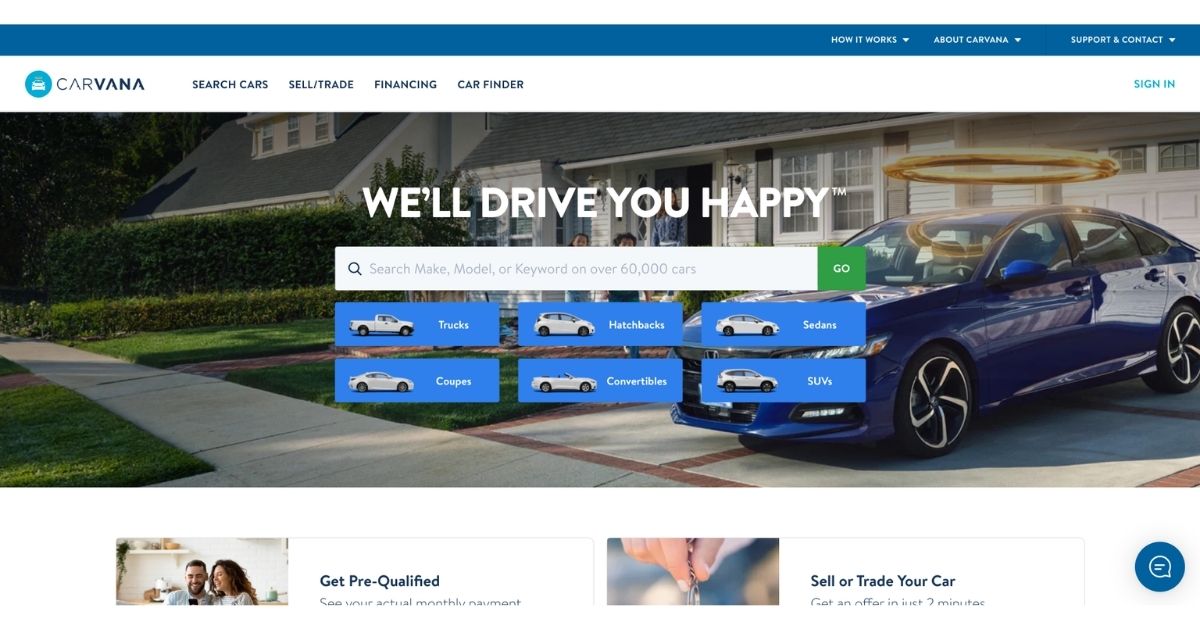In this horizontal left-to-right image, we see a screenshot of a web page from Carvana, accessible via a computer or smart device. 

**Upper Section**:
- The topmost strip is a long rectangular teal banner, prominently featuring the Carvana logo on the upper left.
- On the right side of the teal strip, there are links in white text: "How it Works," "About Carvana," and "Support & Contact."

**Navigation Bar**:
- Directly below the teal strip on the left, the main Carvana circular logo is visible.
- The navigation bar includes options such as "Search Car," "Sell/Trade," "Financing," and "Car Finder," along with a "Sign In" button.

**Main Image**:
- The centerpiece of the web page appears to be a background image showcasing a suburban neighborhood with a few houses, hedges, sidewalks, and driveways.
- In the foreground is a blue car adorned with a golden halo, accompanied by the tagline, "We'll Drive You Happy."

**Search and Categories**:
- A prominent search bar invites users to search by "Make, Model, or Keyword" among over 60,000 cars. Adjacent to the search bar is a green "Go" button.
- Below the search bar, a blue box showcases various categories of vehicles: Trucks, Hatchbacks, Sedans, Coupes, Convertibles, and SUVs – each represented with an icon and label.

**Lower Section**:
- The lower portion of the screen features a white background with partially visible features:
  - "Get Pre-Qualified" is accompanied by an image, though part of the description is cut off.
  - Another segment reads "Sell or Trade a Car," also partially obscured.

**Additional Feature**:
- A chat button is located at the bottom right, offering further assistance.

This carefully structured layout ensures easy navigation and access to essential features for prospective car buyers and sellers.